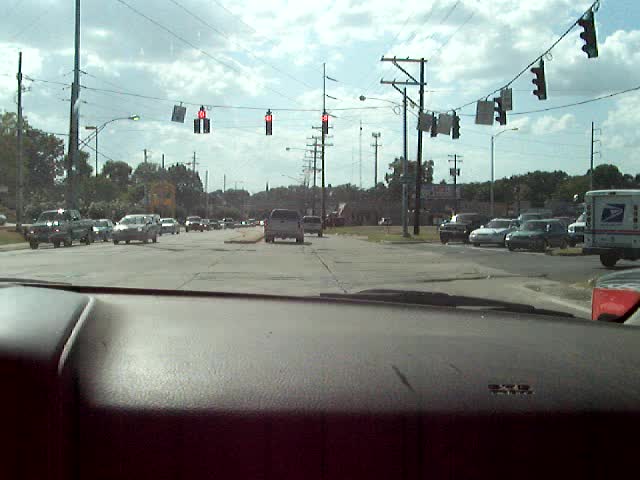A photograph taken from inside a car through the windshield captures the scene ahead. The bottom part of the image reveals a section of the black dashboard. Outside the windshield, a bustling roadway is visible, with numerous cars moving in various directions. Prominently, three traffic lights suspended from power lines show red signals, commanding the vehicles to halt. The road on which the car is driving intersects perpendicularly with another road, where multiple cars are stationary, also waiting at the red lights. In the background, trees line the roads, adding greenery to the urban setting. Above, the sky appears mostly cloudy, with patches of blue peeking through, creating a tranquil yet dynamic atmosphere.